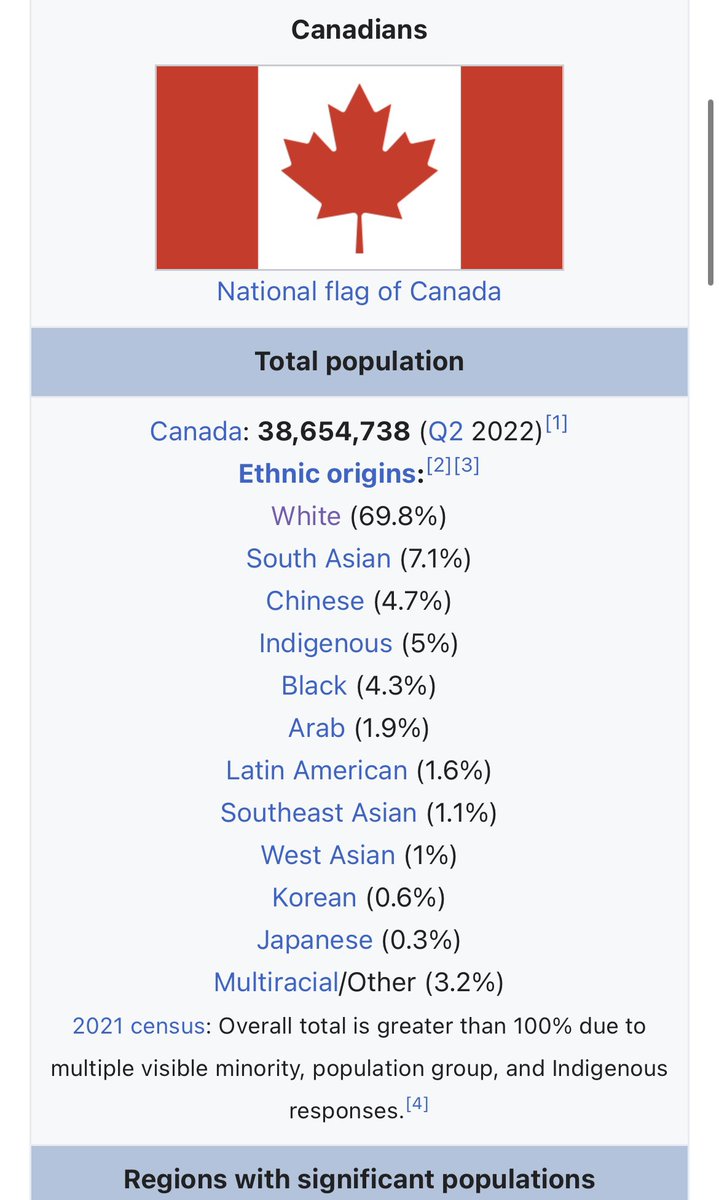The image appears to be a detailed and visually structured segment of a Wikipedia page focused on the demographics of Canadians. It features a vertical layout with the following elements:

- **Header**: At the top, the word "Canadians" is prominently displayed in black.
- **Flag**: Directly beneath the header is the Canadian flag.
- **Flag Description**: Below the flag, in light blue text, it says "National flag of Canada."
- **Total Population**: A light blue bar extends across the page, containing the text "Total population" in black. Beneath this bar, it is stated that Canada has a population of 38,654,738 as of the second quarter of 2022.
- **Ethnic Origins**: Below the population data, another section in blue details various ethnic demographics: 
  - White: 69.8%
  - South Asian: 7.1%
  - Chinese: 4.7%
  - Indigenous: 5%
  - Black: 4.3%
  - Arab: 1.9%
  - Latin American: 1.6%
  - Southeast Asian: 1.1%
  - West Asian: 1%
  - Korean: 0.6%
  - Japanese: 0.3%
  - Multiracial/Other: 3.2%
- **Census Note**: Below the ethnic origins, there is a note in light blue text that reads "2021 census," followed by a black text disclaimer explaining that the overall total may exceed 100% due to multiple visible minority population group and Indigenous responses.
- **Regions with Significant Populations**: Finally, a blue banner states "Regions with significant populations" in black text, although the specific content for this section is not provided.

This layout appears against a light blue rectangular background, giving it a clean and organized appearance that aligns with Wikipedia’s typical informational style.